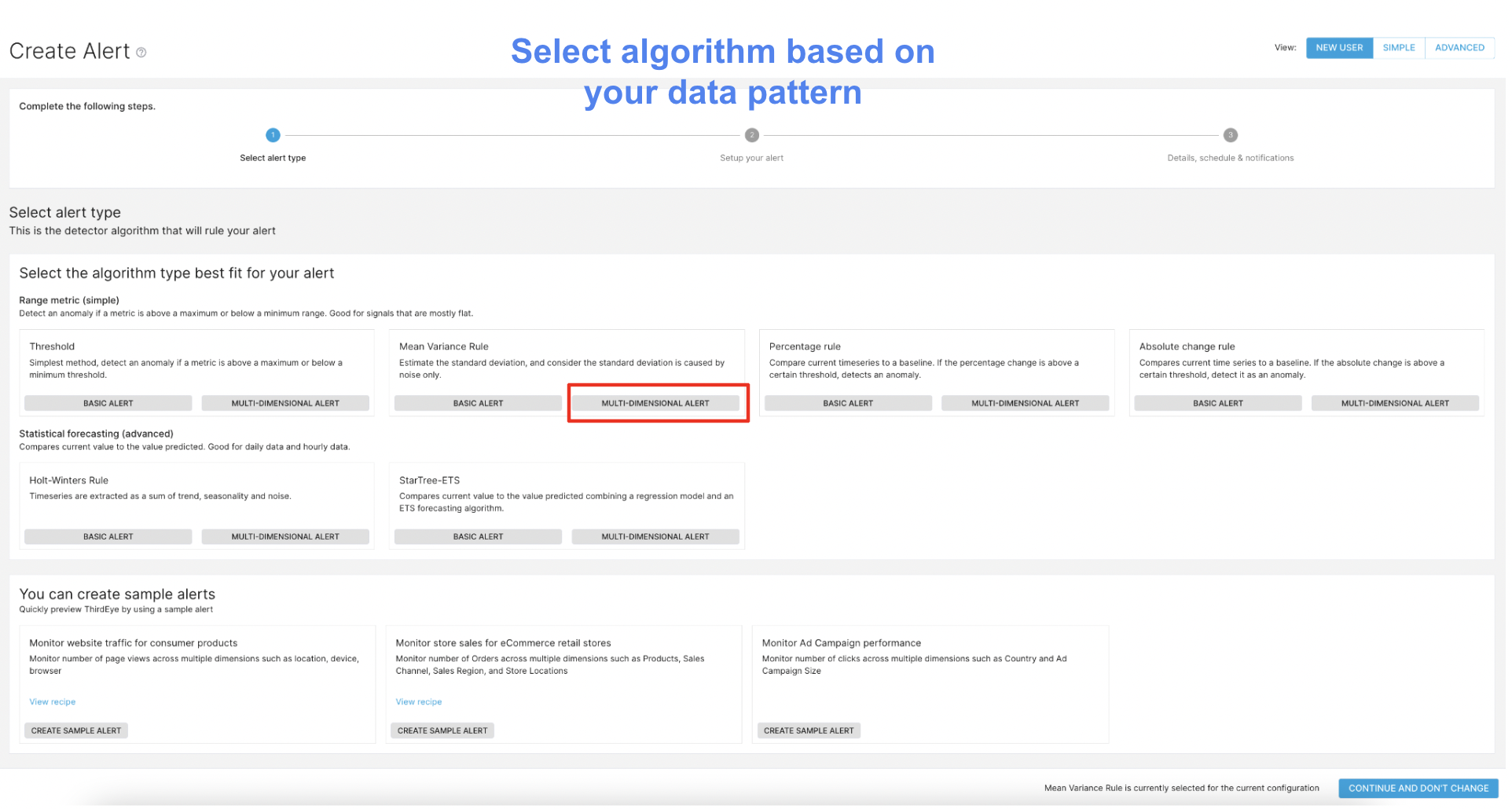In the image with a white background, the top left corner features the text "Create Alert" in black. At the top center, the text "Select algorithm based on your data pattern" is displayed in blue. The top right corner contains several small icons that are too blurry to decipher even when zoomed in. Below these elements, there is a white box occupying the upper portion of the image. Within this box, there is text located on the left side. Adjacent to the text is a horizontal line with three evenly spaced points: one on the left, one in the middle, and one on the right. The left point is marked by a blue circle with small, unreadable text beneath it, while the middle and right points are indicated by gray circles, each also accompanied by unreadable text.

Beneath this section lies a darker gray background with the text "Select alert type" prominently displayed. This area explains that the chosen detector algorithm will influence the alert configuration. Directly below this gray section, a white background reappears, where instructional text reads "Select the algorithm type best fit for your alert." This is accompanied by additional text and two boxes situated at the bottom. One of these boxes is highlighted with a red rectangular shape that appears to have been added via Photoshop.